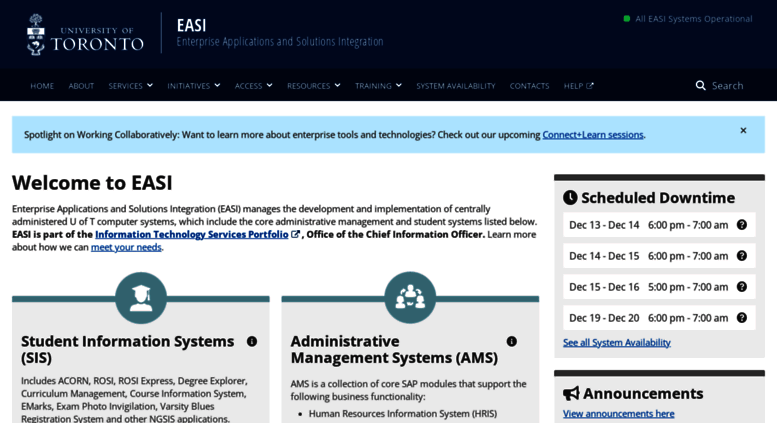The image depicts a section of the University of Toronto's website, specifically focused on Enterprise Applications and Solutions Integration (EASI). The top navigation bar features several options: Home, About, Services, Initiatives, Access—with many of these having drop-down menus—Resources, Training, System Availability, Contacts, and Help, which directs to an external page. Positioned on the upper right is a search bar. This entire top section is styled with a dark blue background and white font.

The main content area of the page is set against a light gray background with black font. A prominent heading, "Welcome to EASI," introduces the section which explains that EASI is responsible for the development and implementation of centrally administered computer systems at the University of Toronto. These systems include core administrative management and student systems essential for campus operations.

On the right side of the page, there is a notice titled "Scheduled Downtime," indicating maintenance periods. The schedule lists several dates in December—13th, 14th, and 15th—highlighting downtime occurrences primarily after 6 p.m., suggesting potential inconvenience for users during these periods.